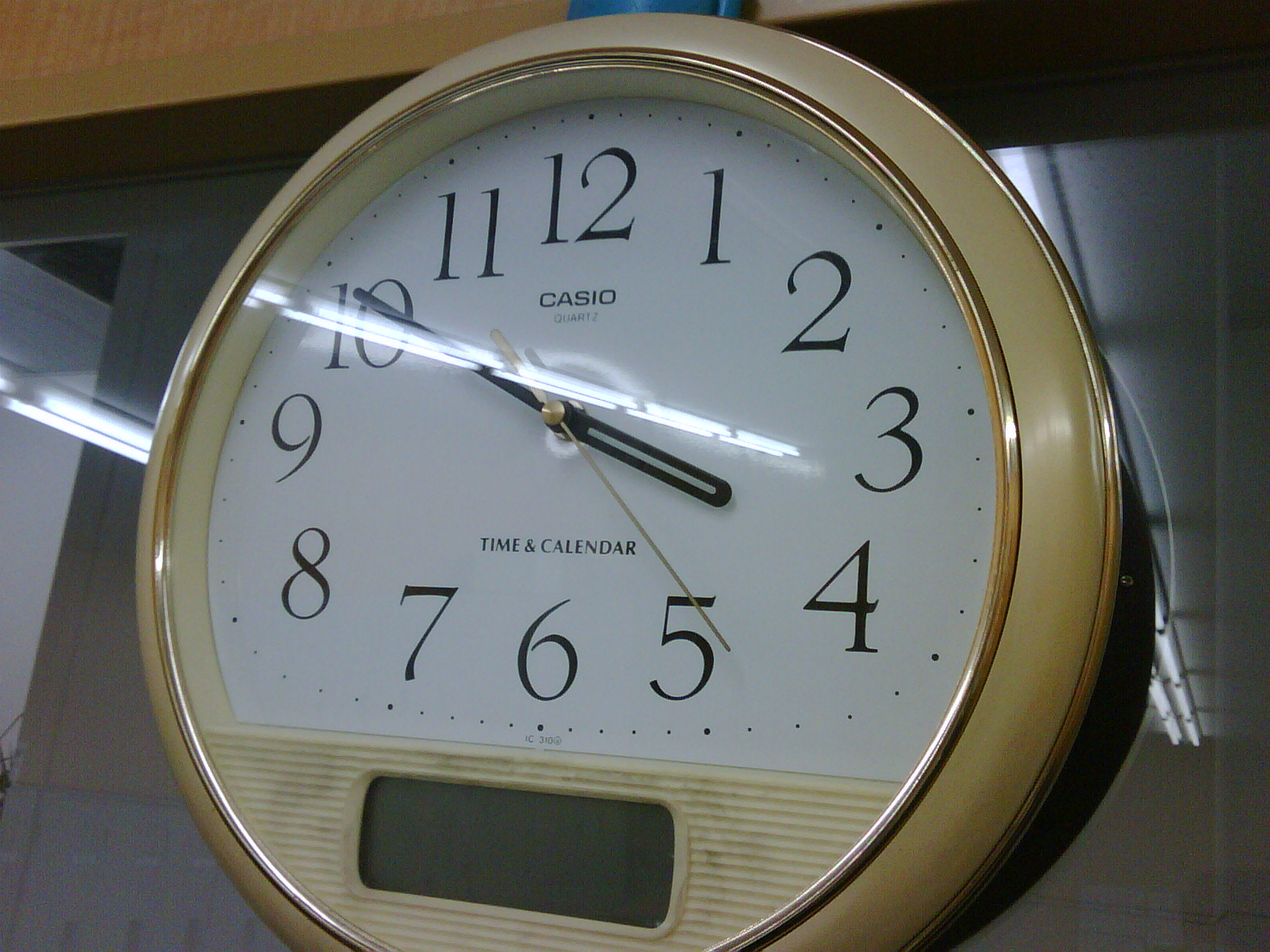This close-up photograph captures a uniquely designed wall clock set against a highly reflective, potentially glass or glossy dark gray background. The clock features a robust, round gold frame that exudes a subtle elegance without being overly shiny. The clock face itself is predominantly white but cleverly integrates a digital panel that occupies the lower quarter, creating a slight squish in the traditional analog display. Despite this adjustment, all standard clock numerals are present. The analog hands indicate the current time as approximately 3:50. The overall composition juxtaposes modern digital elements with classic analog charm against a sleek, reflective surface, enhancing the visual interest of the scene.